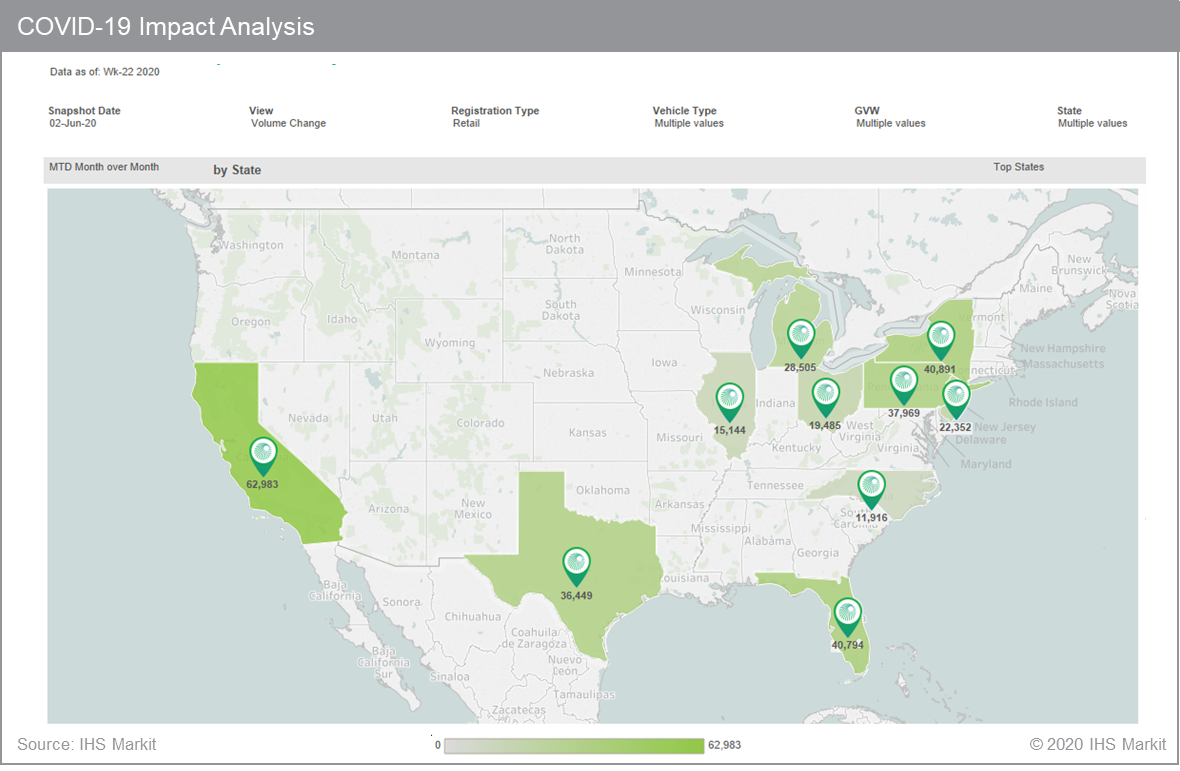The image is a horizontally rectangular frame with a thin, very fine gray border surrounding it. At the top, there is a medium gray horizontal banner. Within this banner, positioned at the top left in white text, are the words "COVID-19 Impact Analysis." Below this on the white background, the text reads "Data as of Week 22, 2020." Further down, horizontally aligned, are several key data points: "Snapshot Date: 2nd June 2020," "View: Volume Change," "Registration Type: Retail," "Vehicle Type: Multiple Values," "GVW: Multiple Values," and "State: Multiple Values."

Directly beneath, there is a narrow, light gray horizontal banner displaying "MTB (Month Over Month)" and indicating the selection option is "By State." To the right within this same banner, it says "Top States."

The main part of the image features a detailed map of the United States, with various states highlighted in green, showcasing their COVID-19 data. Some of the highlighted states include California, Texas, North Carolina, New York, and Pennsylvania.